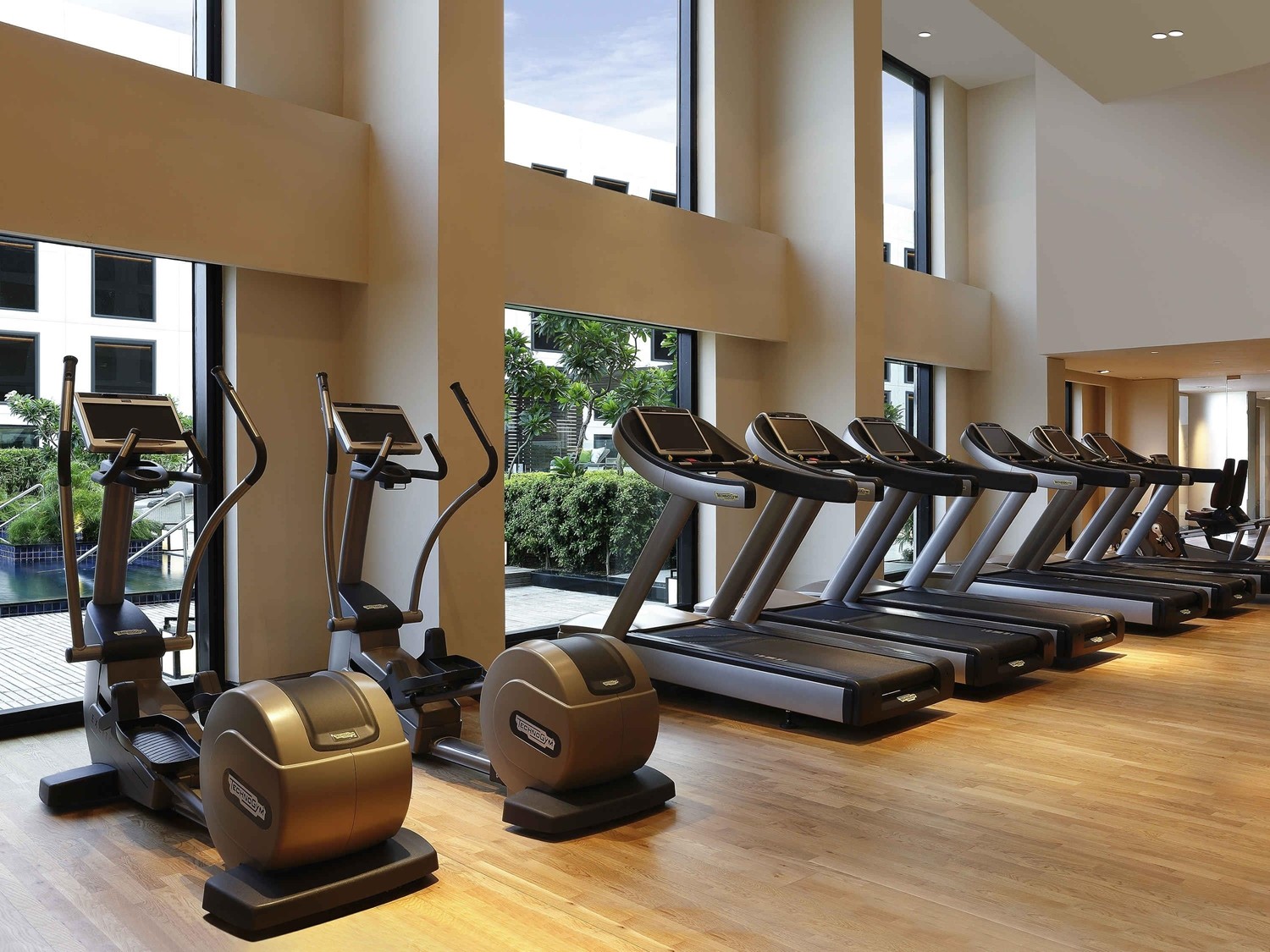The photograph captures a segment of a gym, potentially located within an apartment complex or hotel, distinguished by its inviting decor and thoughtful design. The gym features cream-colored walls adorned with large windows that flood the room with natural light. The windows are strategically positioned in two rows; three large panes align the bottom, separated by a substantial concrete girder, with another row of three topping the entire expanse of one wall.

The gym is equipped with six treadmills arranged on a stunning honey-colored hardwood floor, all aligned to provide users with an engaging view of a courtyard that includes a refreshing pool, lush green bushes, and small trees. Additionally, two elliptical machines are also positioned to face the picturesque outdoor scenery, allowing exercisers to enjoy the serene environment or observe activities by the pool while working out.

On the right-hand side of the image, there is a glimpse into an adjacent corridor, hinting at the spaciousness and connectivity of the facility. The overall ambiance of the gym is both modern and welcoming, designed to enhance the workout experience with both functionality and aesthetic appeal.